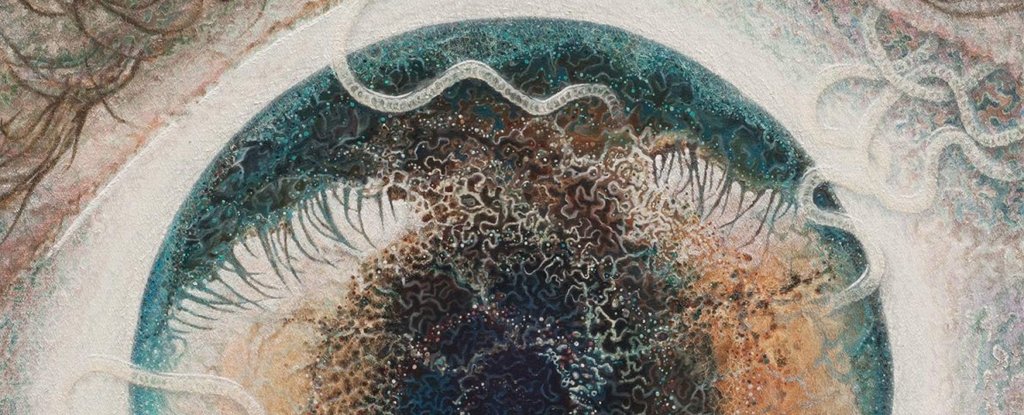The image depicts an incredibly detailed, hyper-realistic illustration of a human eye rendered in graphite or colored pencil. The close-up view focuses on a blue-green eye with a dark brown-black pupil that blends seamlessly into a lighter orange-brown hue. The artist's meticulous attention to detail is evident in the reflection of delicate eyelashes on the eye's surface, as well as the intricate texture of the iris. Surrounding the eye are eerie, milky-white, worm-like figures that appear to be invading the sclera and cornea, lending a surreal and disturbing quality to the artwork. The translucent worms are primarily clustered around the top right corner of the eye, with some starting to burrow into the iris and another emerging from the bottom. This uncanny amalgamation of hyper-realism and abstract horror showcases the artist's exceptional skill while evoking a sense of discomfort and fascination.